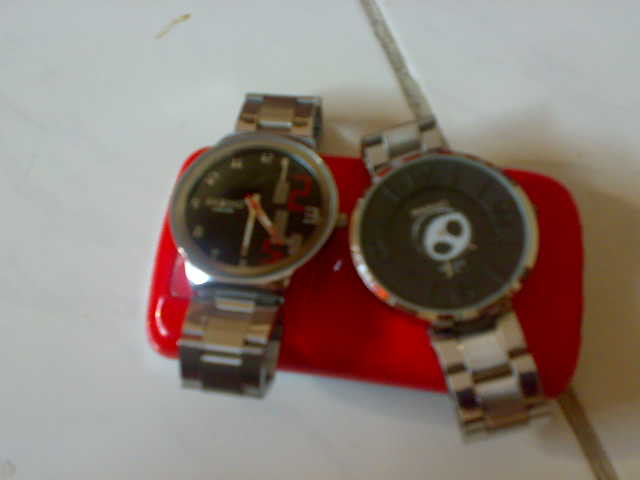This image showcases two watches placed on a polished white counter. The watches are elevated on a striking red platform that holds them securely in place. The timepiece on the left features a modern design with regular numerals; the numbers 2, 3, 5, and 12 are prominently displayed in a large red font, while the other numbers are smaller and white. The watch hands indicate that the current time is approximately 4:30. The companion watch, though harder to discern as it utilizes Roman numerals, complements the first with a similar aesthetic. Both watches boast sleek, silver metallic bands, emphasizing a sophisticated and contemporary style.